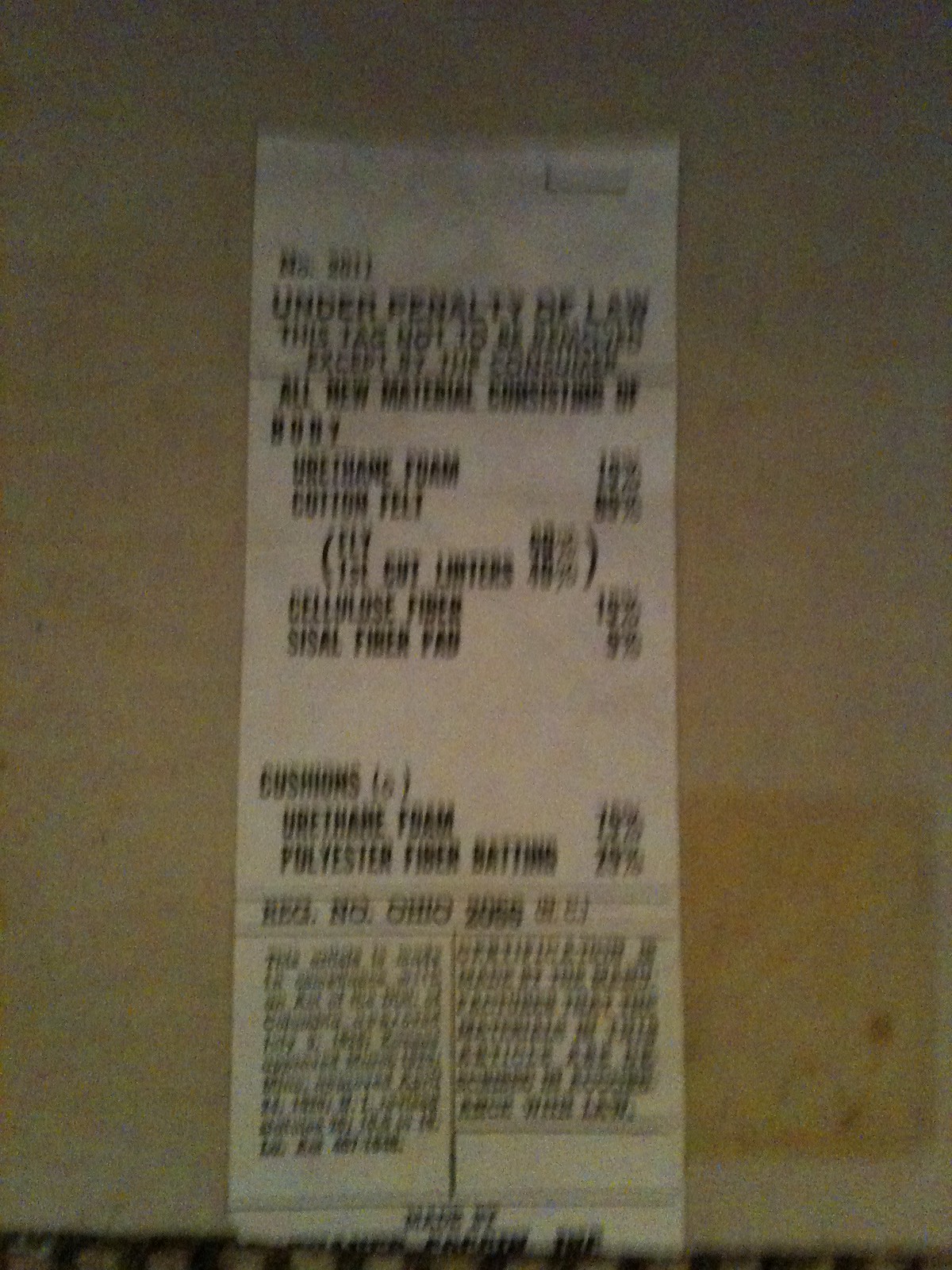The image depicts a highly blurred and difficult-to-read white rectangular tag on a piece of furniture or a mattress, set against a beige background. The tag features black print and is commonly found on items like pillows. The most readable part of the text states: "Under penalty of law, this tag is not to be removed except by the consumer." It also mentions that the item contains materials such as cotton felt and urethane foam, although the rest of the words are obscured. Additionally, parts of the tag include a "register number Ohio" and other numbers, with further smaller and blurred writing underneath.